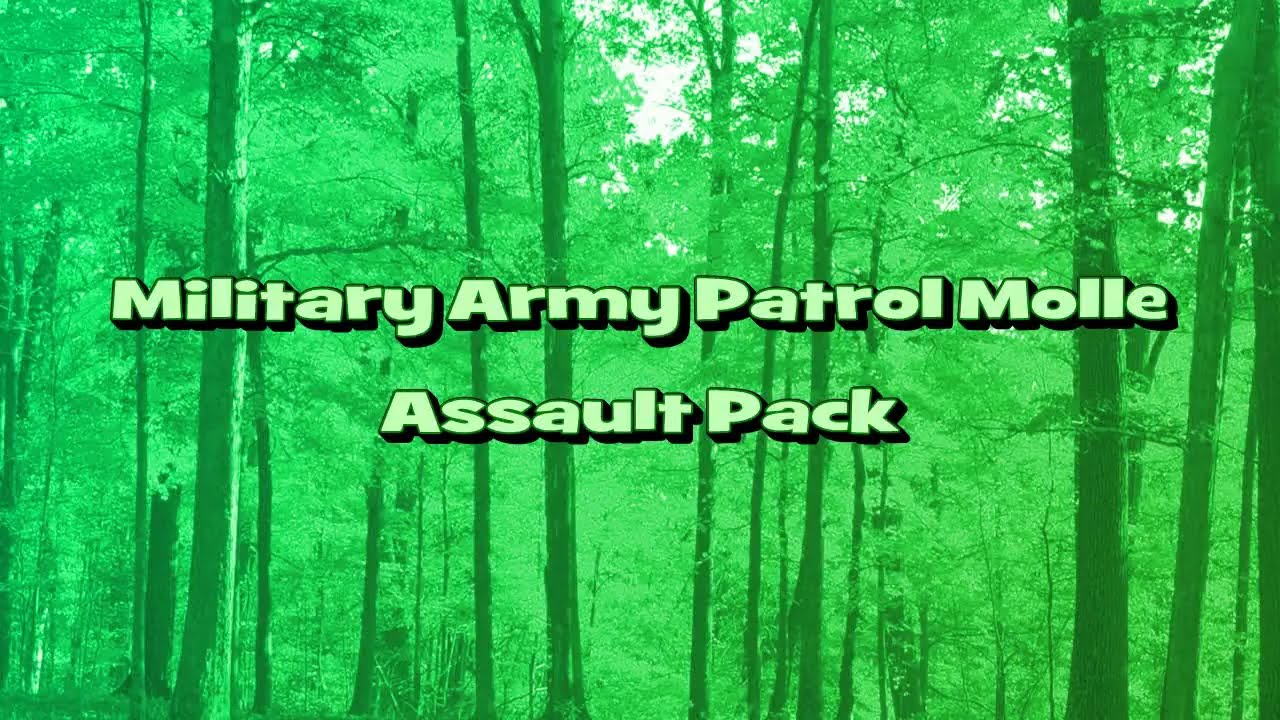The image depicts a forest scene that appears to be viewed through a green filter, giving it an almost fluorescent, neon green hue. The tall, skinny tree trunks dominate the scenery, their greenish-brown bark accentuated with green highlights. Hazy patches in the canopy where leaves should be add to the surreal effect, and some patches of a whitish-gray sky are faintly visible through the dense foliage.

Superimposed in the center of the image is bold, white text outlined in black, creating a three-dimensional effect. The text reads: 

"Military Space Army Space Patrol Space M-O-L-L-E" 

Below this, another line of text reads: 

"Assault Space Pack." 

The text is highly legible due to its mint-green color and the black outline, which contrasts sharply with the vivid green forest background. The overall effect is striking and somewhat otherworldly, emphasizing the unnatural lighting that bathes the entire forest scene.